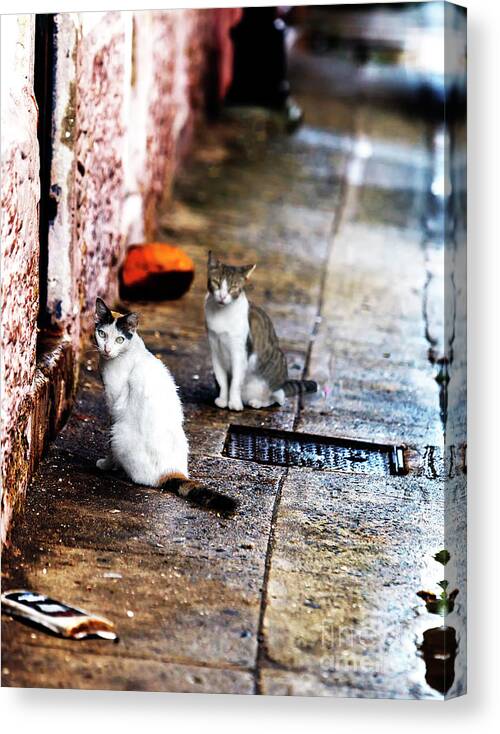In a cluttered, grimy alleyway filled with various pieces of litter, two cats stand near a small sewer grate. The cement ground is visibly wet, with a shiny texture that suggests the presence of water or oil, and is mottled with shades of brown, black, and gray. The first cat, primarily white with a bushy black tail and distinctive black spots over its eyes, has a pink nose and light-colored eyes. It has black ears and some brown on the top of its head. This cat is looking over its shoulder with a somewhat scared expression. Behind it stands the second cat, which has a white chest and stomach but is marked by a black stripe and brown fur on its back and the top of its head. This cat also has a striped black tail and white markings on its nose, with its eyes appearing squinted. Both cats are framed against the backdrop of a light-colored wall and are gazing directly at the camera, emanating a sense of wariness. The image blurs into the distance, adding to the gritty and aged atmosphere of the alley.